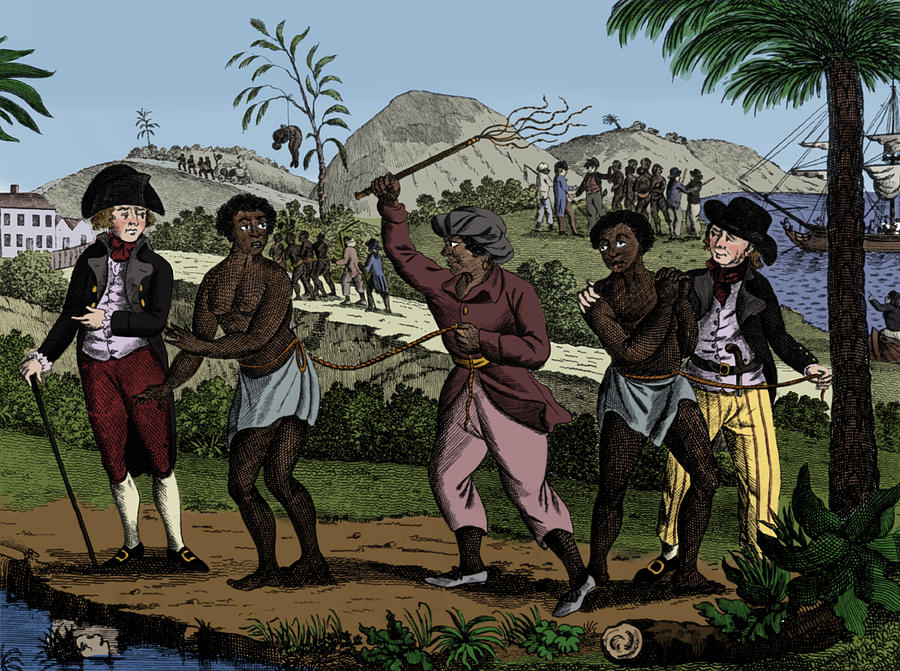The illustration presents a highly disturbing and evocative scene of British colonial soldiers orchestrating the forced transport of enslaved individuals onto ships. In the foreground, several African men, depicted with darker skin and dressed in blue loincloths, are bound with ropes around their stomachs. One of the enslaved men on the right is forcibly grasped by a white man clad in pinstripe yellow pants, a black jacket, and a black hat, with a gun visibly tucked into his belt. Centrally located in the image is a well-dressed black woman, distinguishable by her switch or broomstick, which she wields while holding a rope attached to one of the slaves. The background reveals the grim context of the scene, with hanging bodies from trees, an array of ships by the waterfront, and scattered rocks. Additional elements include palm trees and verdant surroundings, reinforcing the tropical setting. The entire composition is intricately rendered in a crosshatch style, suggesting it is an illustrated, perhaps stenciled or penciled, piece rather than a traditional painting.